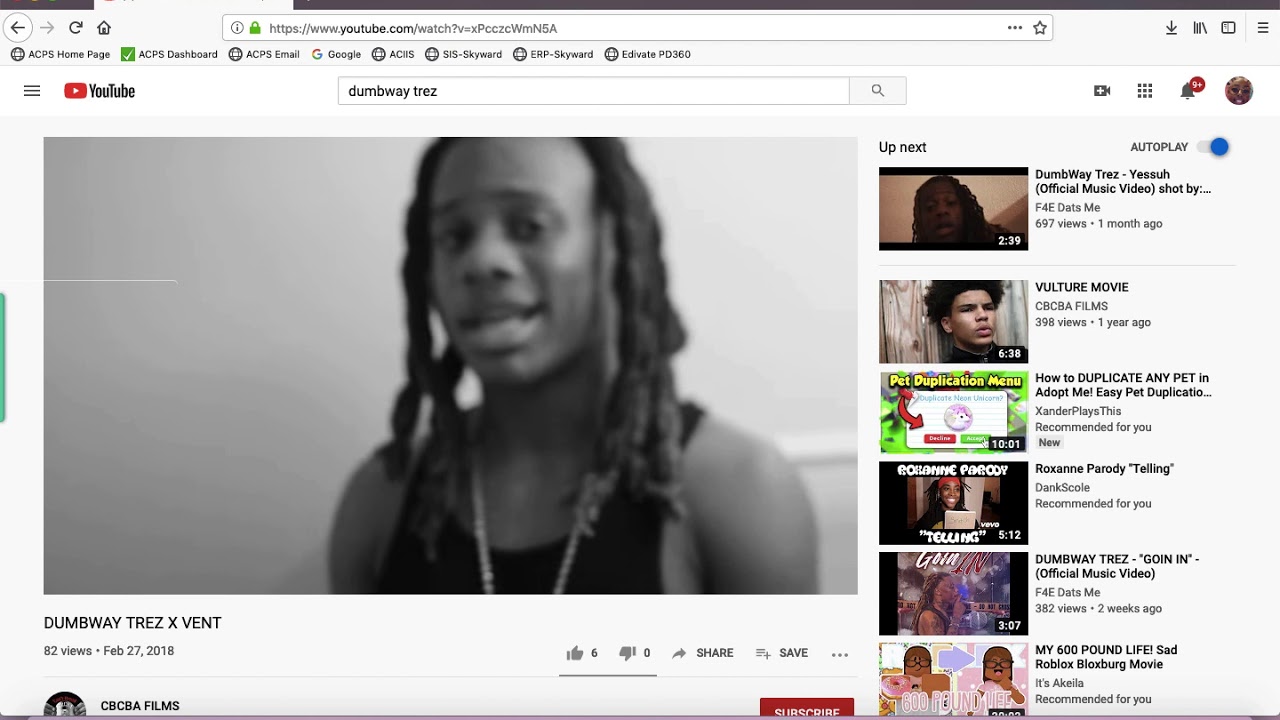The web page depicted in the image is a YouTube results page. The address bar clearly shows "youtube.com." At the bottom of the page, the YouTube logo is situated next to a hamburger menu icon. In the search bar, the term "dumb way trays" is entered. 

To the right of the search bar, there are several icons lined up: a camera, a square composed of nine smaller boxes, a notifications bell, and a user's profile photo. The main content area of the page features a still image of an African American rapper with dreadlocks, wearing a chain and a black wifebeater. Below the image, the text reads: "Dumb Dumb Boy Tres X Vent," with 82 views, dated February 27, 2018.

To the right of the video title, there are icons showing six thumbs up, zero thumbs down, a share button, and a save button. The page also includes an option to subscribe to the channel. Below this, there is a list of upcoming videos, with titles such as "Dumb Way Tray Official Video," "The Movie Vulture," "How to Duplicate Any Pet in Adopt Me," "Roxanne Parody," "Telling Dumb Way Trays Again," "Going In Official Music Video," and "My Six of the Pound Life," a "Roblox Bloxburg" movie.